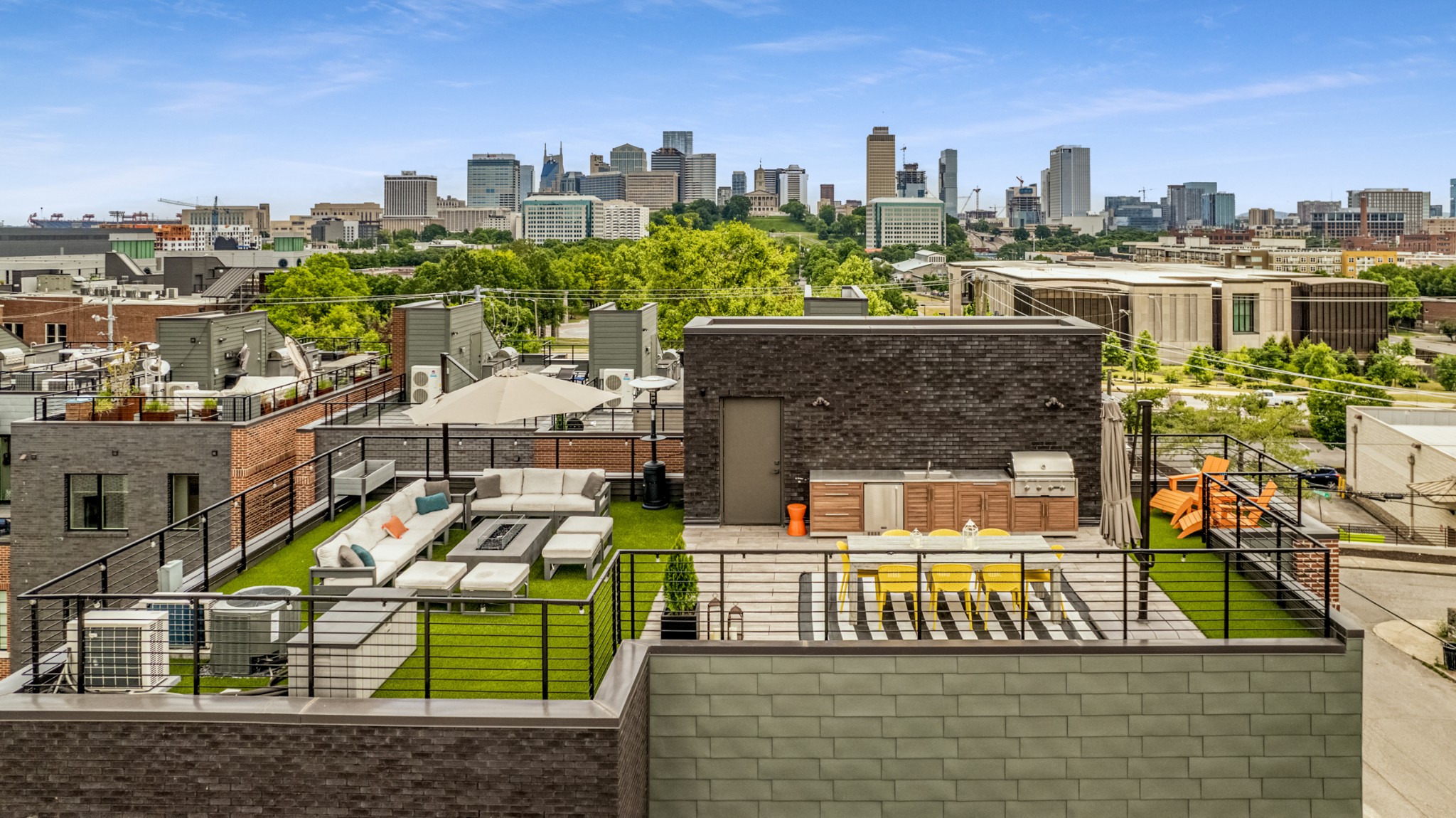This image captures a detailed rooftop living space perched atop an apartment complex in a bustling city. The main rooftop space, covered with astroturf to simulate grass, features a well-organized outdoor seating area. In the center, two couches, surrounding a fire table with a sun canopy overhead, invite relaxation. Ottomans are strategically placed around the fire table, while planters accentuate the corners of the space. A utility section is marked by the presence of air conditioning units. Adjacent to the seating area, a fully equipped outdoor kitchen includes a grill, refrigerator, sink, and cabinetry, all backed by a dark brick wall with an access door. An additional dining area with a table and yellow chairs completes the setup. The rooftop is surrounded by an industrial-looking fence, adding a touch of safety and style. In the foreground, similar rooftop setups can be seen on neighboring buildings. The expansive background showcases a vibrant cityscape featuring tall buildings and skyscrapers set against a blue sky dappled with light clouds, while patches of greenery and residential complexes create a textured urban landscape.